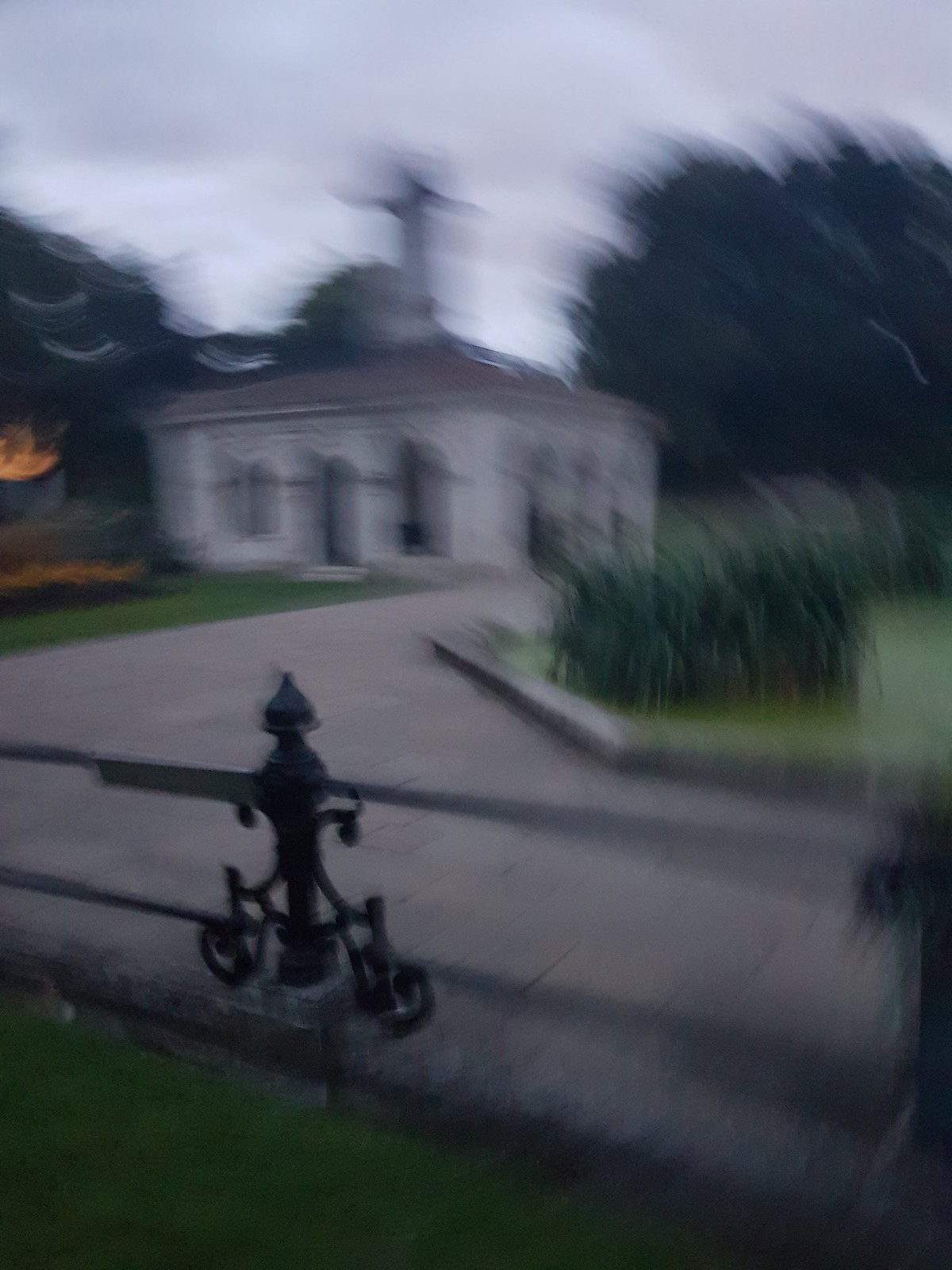In this photograph, taken outdoors, we observe a scene captured with considerable motion blur, creating a spinning effect that makes it difficult to discern details clearly. Central to the image is a tall, white building that evokes the appearance of a historical or religious structure, potentially a mausoleum or a small church. The building features high archways and arched windows, with something indistinct perched atop it. In the foreground, a stone sidewalk stretches past the building, bordered by patches of grass adorned with plants or flowers. Further in the background, we glimpse a few trees, adding to the natural ambiance. Despite the blurriness of the photo, the overall setting suggests a quaint, possibly tranquil, outdoor environment without any textual information provided.